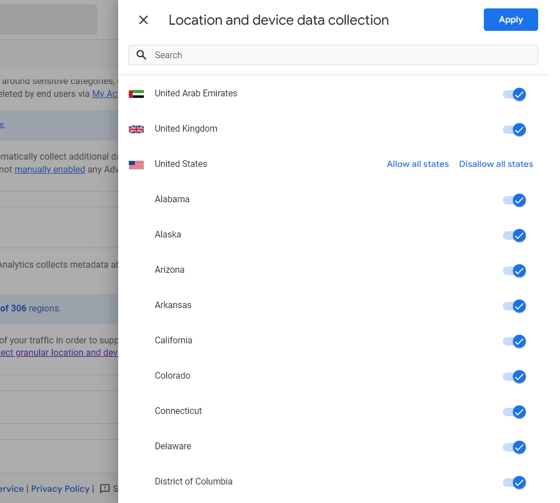A screenshot of a settings interface for location and device data collection. At the top, the header reads "Location and Device Data Collection." To the right of this header is a blue "Apply" button. Below the header is a search bar, and beneath it, a list of locations: "United Arab Emirates, United Kingdom, United States, Alabama, Alaska, Arizona, Arkansas, California, Colorado, Connecticut, Delaware, and District of Columbia." Each location has a corresponding toggle switch to its right. These switches have a light blue bar and a dark blue circle with a white check mark inside, indicating that all options are currently toggled on.